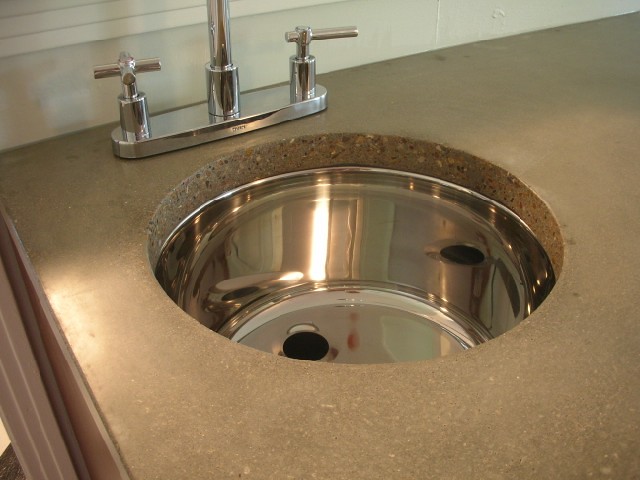This close-up, catalog-quality photo captures a meticulously lit kitchen countertop. The countertop appears to be a composite material, possibly Corian, showcasing a brownish-gray hue accented with black flecks and white chunks. The perspective allows us to appreciate the countertop's substantial thickness, revealing a circular cutaway where a sleek, stainless steel sink is seamlessly integrated. The sink, set below the counter surface, highlights the clean cutaway edge, emphasizing the countertop’s impressive inch-thick build. 

The perfectly round sink boasts a shiny, reflective finish, with a visible black drain hole positioned slightly off-center due to the angled view. Mounted directly behind the sink is a modern, chrome-plated faucet assembly. The faucet features a sturdy base plate and contemporary handles which stand upright, culminating in unique cross-tops with extended arms for easy operation. While the photo cuts off midway up the spout, one can discern that the spout has a prominent arc design intended to extend over the sink for optimal use. 

In the background, the image includes a segment of a tile backsplash, subtly framed by what appears to be white lateral trim. This trim might be part of a mirror frame or decorative molding, adding an elegant touch to the overall kitchen design. 

Overall, this detailed snapshot highlights the combination of modern utility and aesthetic appeal in a high-end kitchen setup.